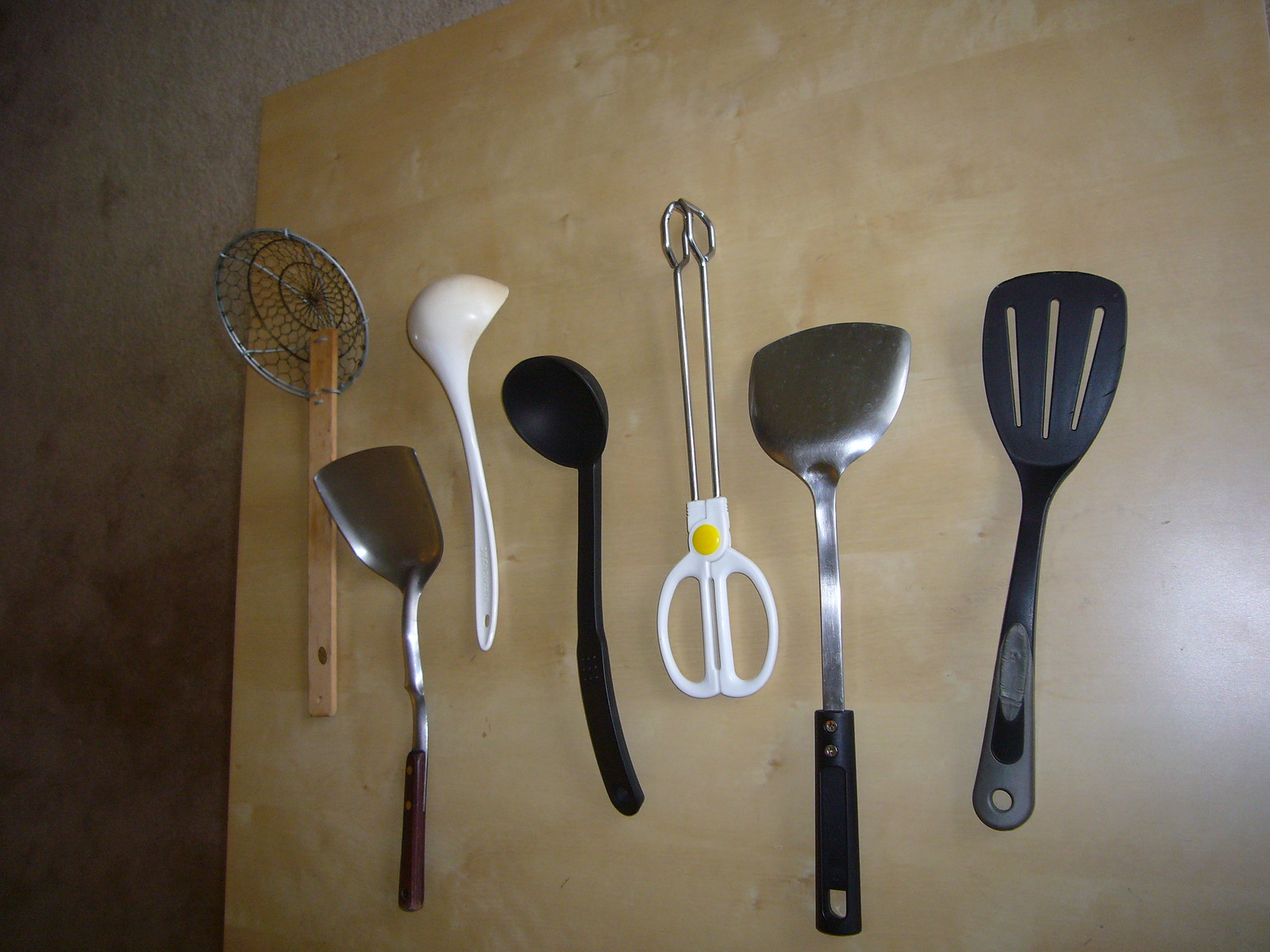The photograph captures a light pine-colored table from an aerial view, occupying three-quarters of the frame. The remaining quarter on the left edge reveals a floor of rich, dark brown, resembling mahogany. Arranged neatly on the table are seven kitchen utensils, listed from left to right. First, there's a handheld strainer with a metal sieve and a wooden handle, possibly for poaching eggs. Next, a ladle with a bent wooden handle is positioned beside a white plastic scoop, commonly used for serving fruit salad, soup, or regular salad. Following these is a similar scoop in black plastic. A set of tongs with silver arms and white handles features a yellow circle clasp. A metal spatula with a brown handle, designed for flipping food, is next. Finally, a black turner with an all-black plastic body completes the lineup. Each item is carefully placed, highlighting their design and utility.